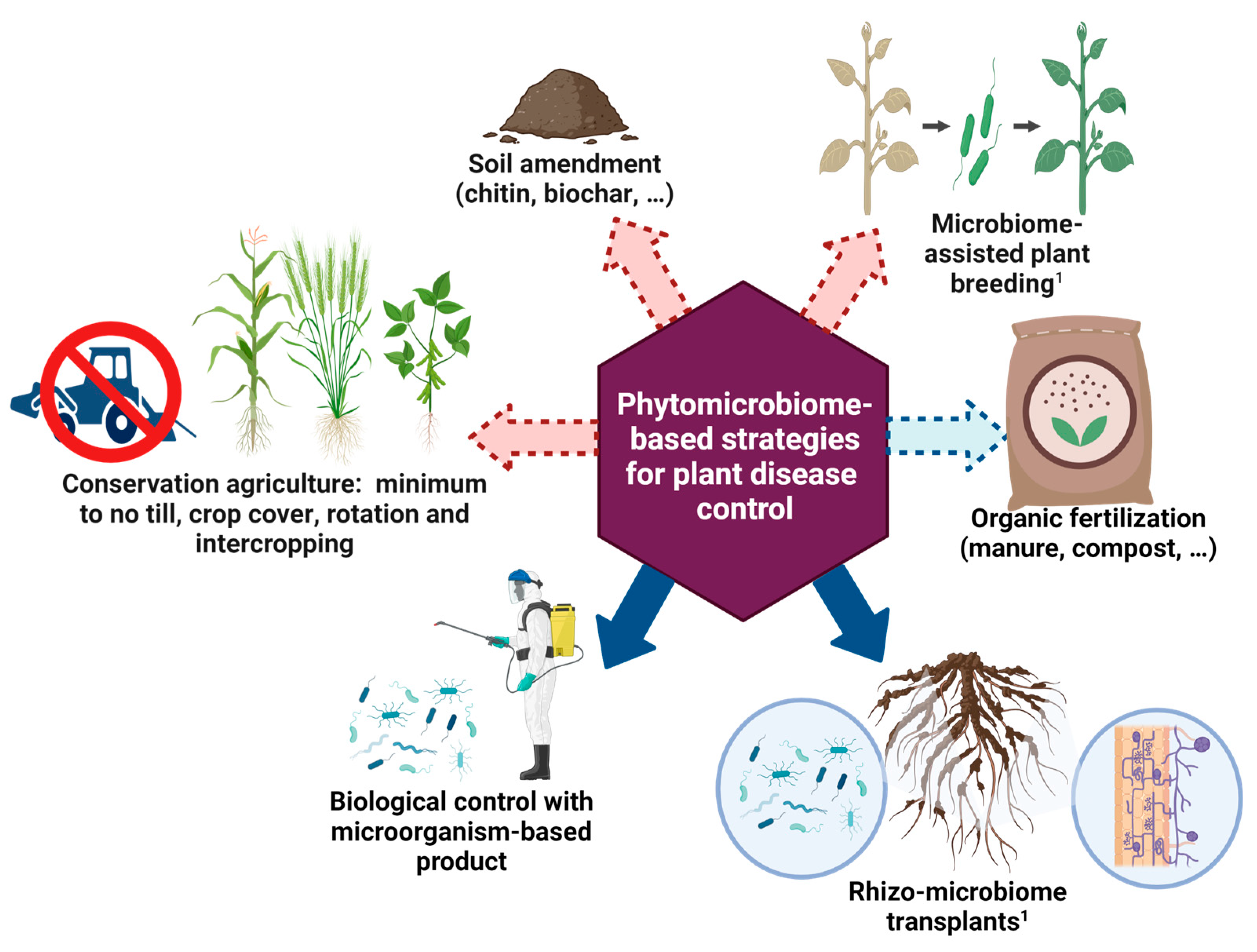The image features a detailed and colorful diagram with a white background, illustrating various strategies for plant disease control through the phytomicrobiome approach. At the center of the diagram is a burgundy hexagon with white text reading "Phytomicrobiome-Based Strategies for Plant Disease Control." Arrows extend from the hexagon in six different directions, each pointing to a specific strategy accompanied by illustrative images.

Starting from approximately one o'clock and moving clockwise:

1. **Microbiome-Assisted Plant Breeding:** This section depicts leafy plants transitioning from beige to green, illustrating the process of enhancing plant genetics through microbiome assistance.
   
2. **Organic Fertilization:** Illustrated with a bag of manure and compost, this part highlights the use of organic materials to enrich soil health.

3. **Rhizomicrobiome Transplants:** Featuring a detailed root system with microbiome cells, this strategy focuses on transplanting beneficial root-associated microbiota to fight plant diseases.

4. **Biological Control with Microorganism-Based Products:** A person in safety gear is seen spraying a treatment, representing the use of microbes to control pathogens.

5. **Conservation Agriculture:** Depicted with three plants and a blue tractor crossed out, this section outlines methods such as minimum to no-till farming, crop cover rotation, and intercropping to maintain soil health and reduce disease incidence.

6. **Soil Amendments:** Shown as a brown mound of soil, this strategy involves enriching the soil with substances like chitin and biochar to improve its structure and fertility.

Each strategy is precisely illustrated, making the diagram not only informative but visually engaging as well.